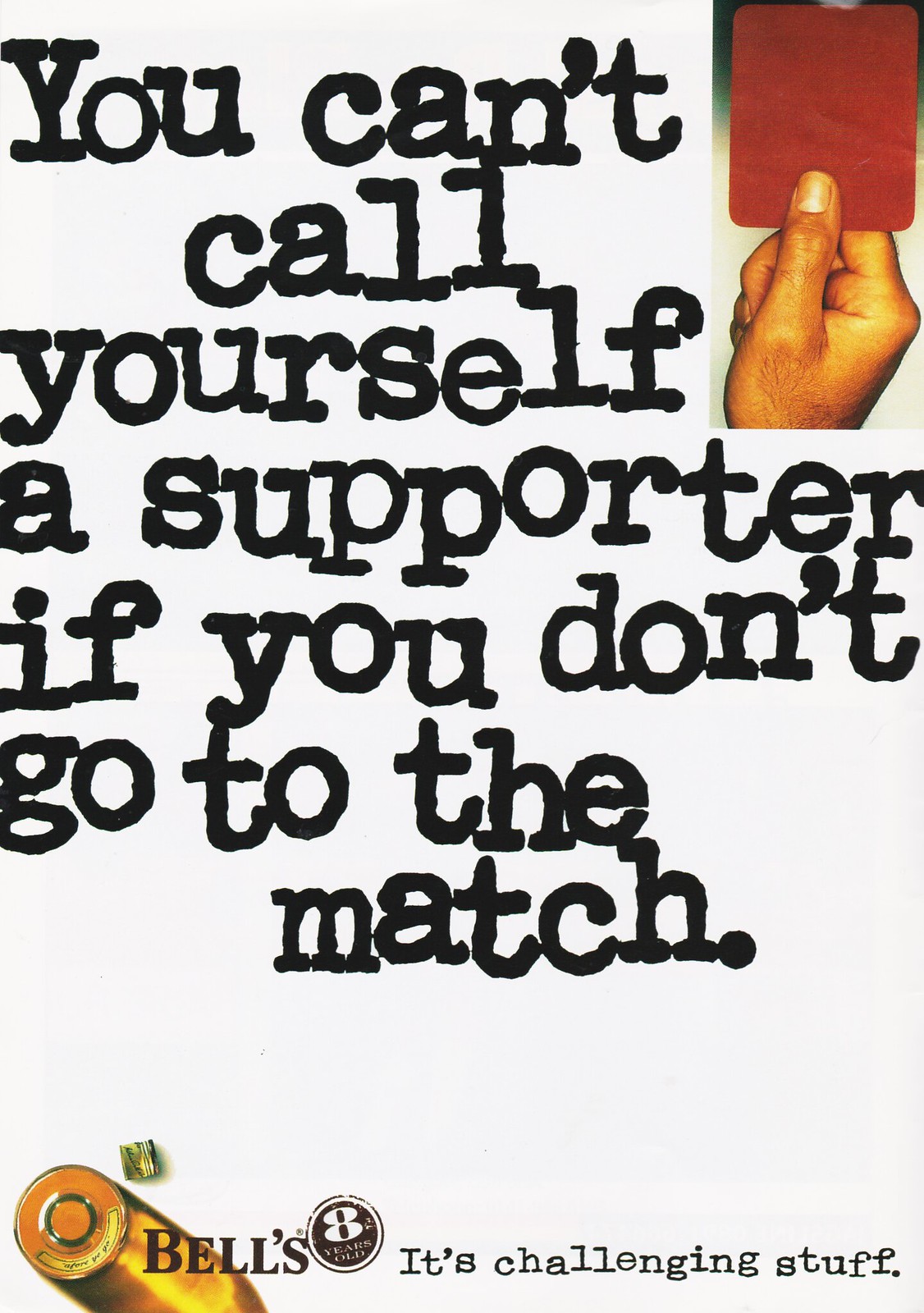This image is a color photograph blended with graphic design and typography, set against a white background in portrait orientation. Dominating the center of the composition is bold, typewriter-style text that reads, "You can't call yourself a supporter if you don't go to the match." In the top right corner, a hand is prominently featured holding a red rectangular card. Towards the bottom left, a logo for "Bells" is displayed, accompanied by the text "8 years old," with an illustration of a golden beverage glass situated behind it, and the tagline "It's challenging stuff" appearing just below. The colors in the image include gray, black, red, tan, green, and yellow, with black textual information providing a stark contrast to the white background. The overall style and setting suggest that this is a sports-related advertisement, possibly promoting a product called Bells.